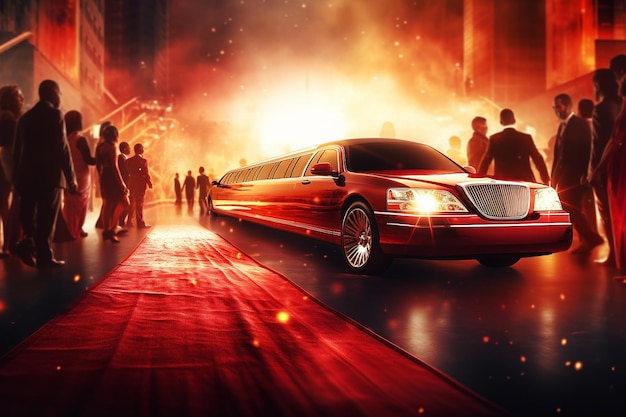The image depicts a vibrant scene that appears to be AI-generated, featuring a striking red stretch limousine prominently positioned on the right-hand side of the composition. The vehicle's headlights are illuminated, casting a bright yellow glow. The limousine is adjacent to a long, luxurious red carpet that extends from the foreground to the background of the image. Numerous people, both men and women, are gathered around the vehicle, all dressed in formal attire such as suits, ties, and elegant dresses, suggesting a high-profile event or glamorous gathering.

On the right side of the limousine, there is a group of men in suits, while the left side features both men and women in fancy clothing. Towards the back of the limousine, as well as near the front driver's side, people are also assembled. The background showcases a tall building to the left and an intense light source coupled with billowing white smoke, creating a dramatic and almost theatrical atmosphere. This light and smoke give an impression of a fiery explosion, although it is likely intended to be a dazzling display of light and sparkle, enhancing the luxurious and opulent feel of the scene.